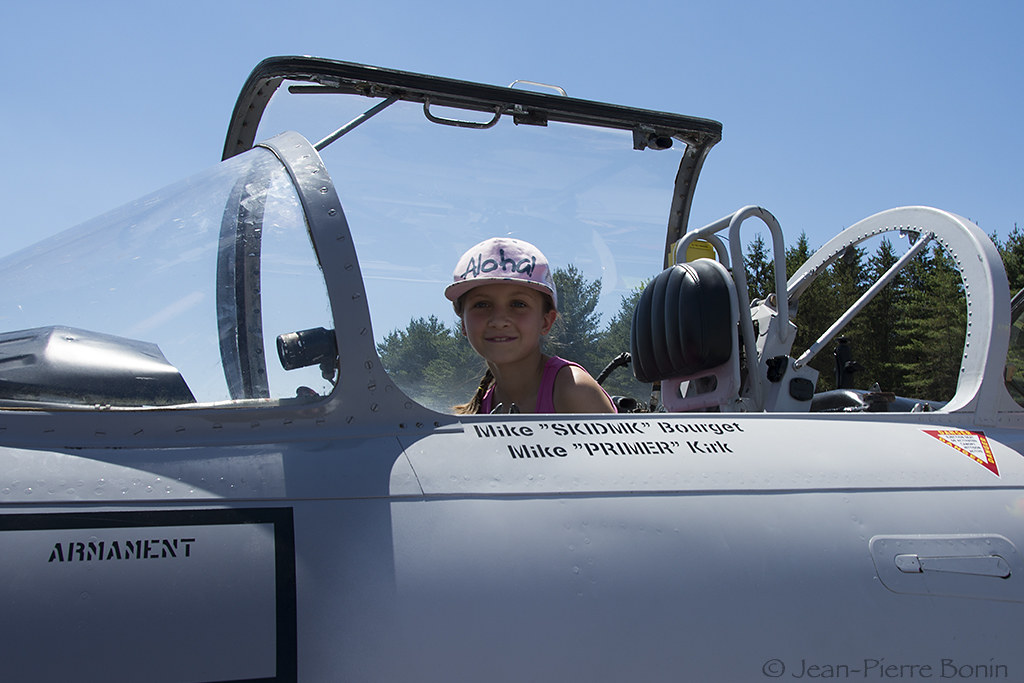In this vibrant, full-color outdoor photograph taken on a bright, sunny day, a young girl, appearing to be between 5 and 8 years old, is the focal point as she sits inside the open cockpit of a parked fighter jet. The backdrop is a pristine blue sky dotted with a few wispy clouds and a dense line of pine trees. The girl, facing the camera with a slight smile, wears a pink baseball cap emblazoned with "Aloha" and a purple tank top, her hair pulled back in a ponytail. The jet itself has a bluish-grayish hue, and inscriptions near the canopy read "Mike 'Skidmark' Borget" and "Mike 'Primer' Kirk," likely indicating the names of the pilot and co-pilot or additional crew members. Another name, "Armin Johnson," is also visible on the side of the aircraft. In the bottom right-hand corner of the image, a watermark credits Jean Pirie Bonin Photography.